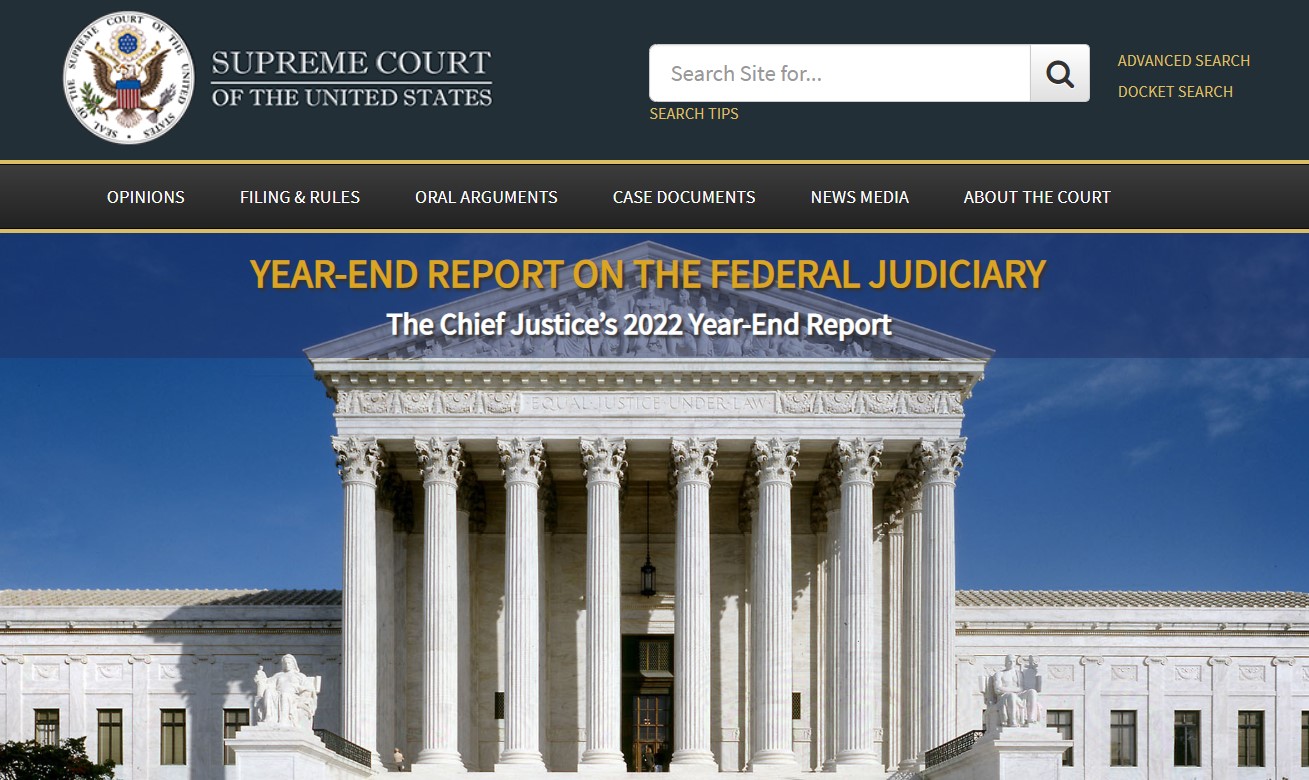A screenshot from a computer displays the homepage of the Supreme Court of the United States. At the top of the page is a dark navy blue banner featuring the Court's majestic seal, which includes an eagle clutching a shield in its talons. This section contains a site search bar labeled “Search Site,” alongside options for “Advanced Search” and “DACA Search.”

Below the banner, there is a brown navigation bar with categories such as "Opinions," "Filings and Rules," "Oral Arguments," "Case Documents," "News Media," and "About the Court." 

Further down, the main content area showcases a striking image of the Supreme Court building's exterior. The photograph captures the iconic architecture against a clear, blue sky. The majestic structure is fronted by eight grand pillars extending down both sides of the entrance, flanked by statues. Text accompanying the image highlights the "Year-End Report on the Federal Judiciary" and links to the Chief Justice's 2022 year-end report. The overall composition of the website conveys the grandeur and significance of the United States Supreme Court.